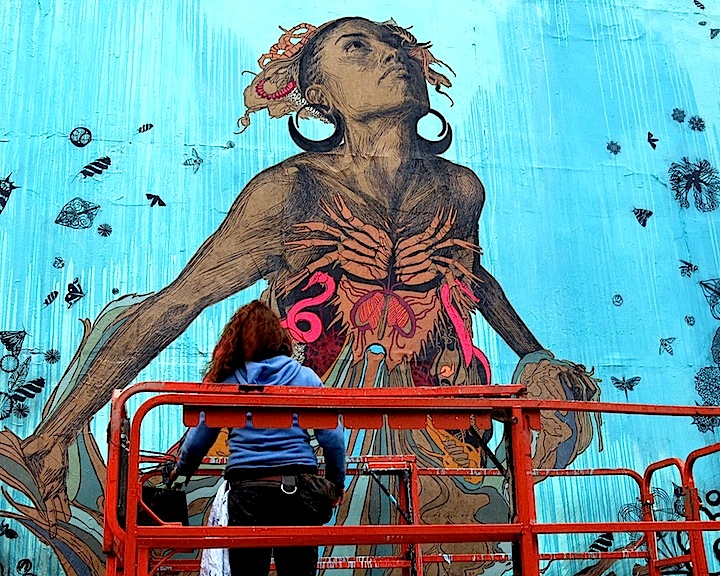The mural, set against a sky blue background with darker blue shades on the sides, is painted on the side of a water tank or aquarium wall. It features an intricate composition of various elements: a butterfly, a bee, a tennis ball, a leaf, dragonflies, and flowers in black. A prominent black woman is the focal point, looking up towards the sky. She wears a tan headdress and large black hoop earrings piercing both her ears. Her dress is elaborate, depicting an orange crab on her chest and an orange, purple, and tan butterfly below it. Her dress is also described as featuring crab legs, a stylized pink snake, and abstract artistic lines. The mural has a surreal quality, with her hair resembling sea creatures and her arms adorned with cloth. In the foreground, a woman, presumably the artist, is seen standing on a piece of scaffolding, positioning herself to continue her work, while she looks up at the mural. The scene is evocative of a Frida Kahlo or Salvador Dali painting, combining realistic human features with fantastical elements.